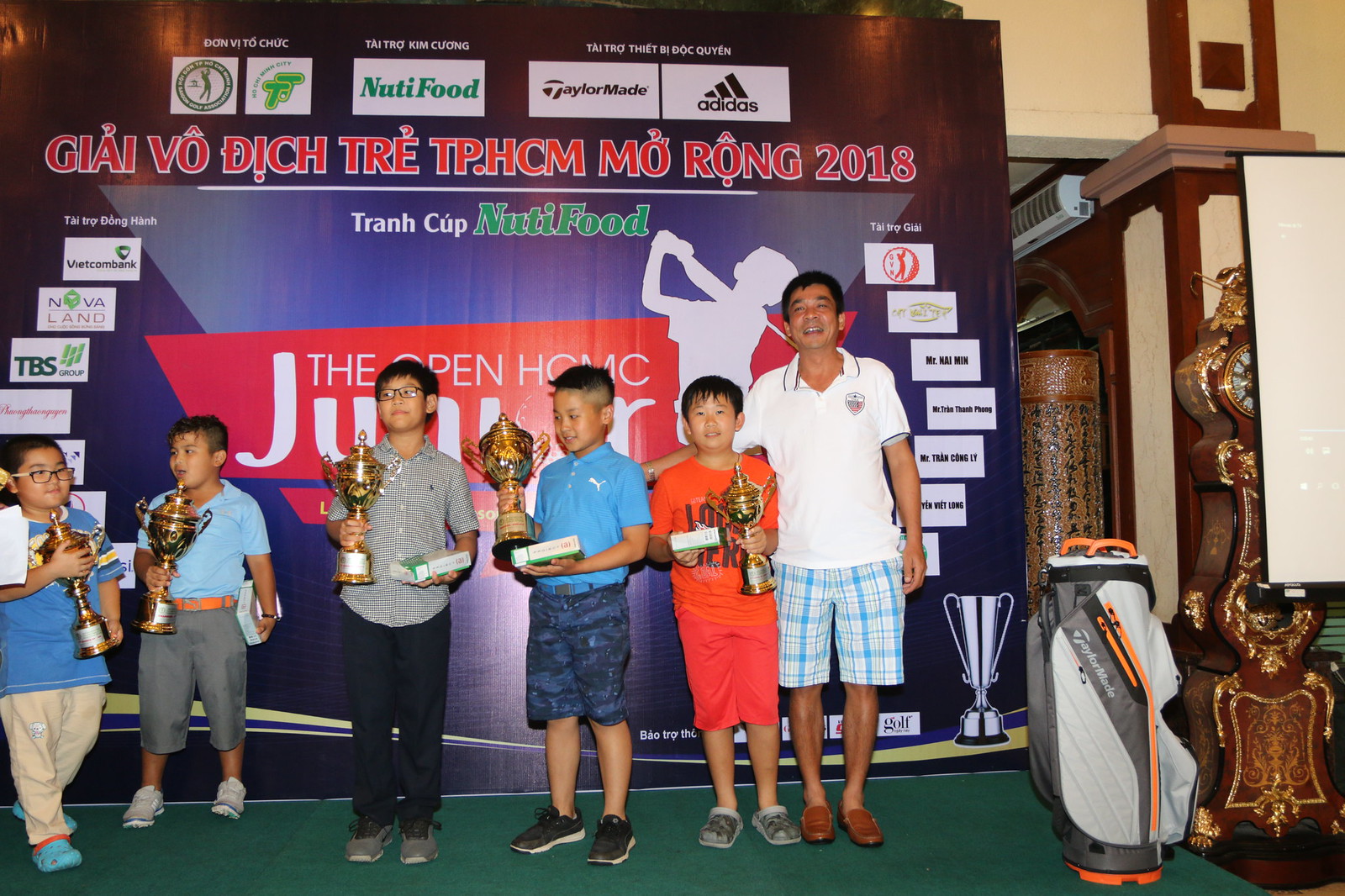This photograph captures a celebratory moment at an awards assembly, likely a golf tournament, held in 2018 and possibly in Vietnam, as suggested by the Vietnamese writing on the backdrop. The scene is set on a stage with six individuals: five young boys and one man. All five boys are proudly holding golden, ornate trophies, which also include a box of some sort, possibly an award or a book. To the far right of the group stands a golf bag, signifying the context of the event. The man, who appears to be close to the boy in the orange t-shirt and red shorts—possibly his father—wears a white polo shirt, blue and white plaid shorts, and loafers.

The boys sport a variety of outfits: the boy next to the man wears an orange t-shirt and red shorts, the boy to his left wears blue shorts, while the next wears a gray plaid shirt and black pants paired with glasses, followed by another boy in a blue shirt and gray shorts. The final child, possibly a girl, wears a blue shirt, tan pants, and glasses.

The backdrop behind them includes multiple advertisements from notable brands such as Adidas, Nutifood, and TaylorMade. Dominating the stage is an orange banner with a white silhouette of a golfer and text suggesting it’s an 'Open' tournament event, further indicated by English snippets like "Junior" and "HCH." The setting and the joyful expressions suggest that the event is a significant and memorable occasion for the participants.